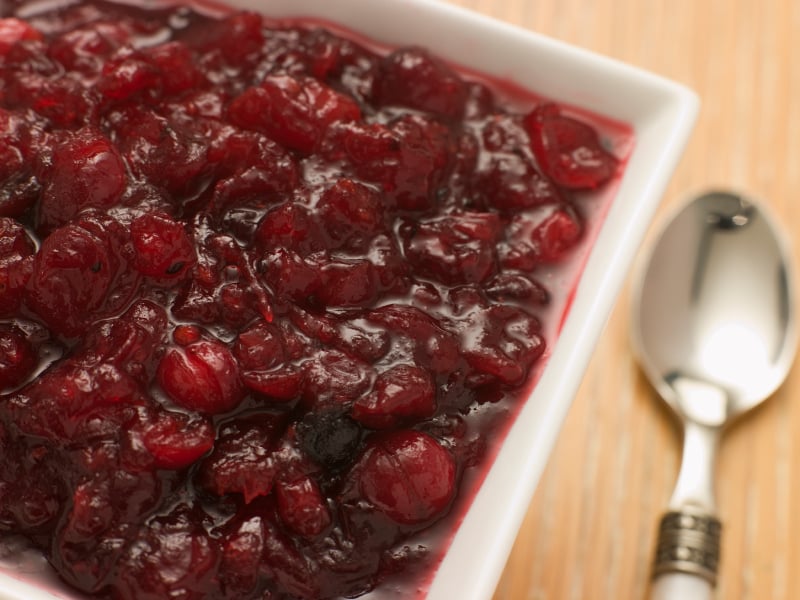The image features a close-up view of a white square bowl containing a chunky red fruit mixture, likely a form of cranberries or pureed strawberries, set atop a light brown wooden surface. The red fruit appears shiny and slightly gelatinous, suggesting a saucy texture. To the right of the bowl is a metallic silver spoon with an ornate ring at the bottom of its head, capturing the light similarly to the glossy fruit and adding a visual contrast to the scene.